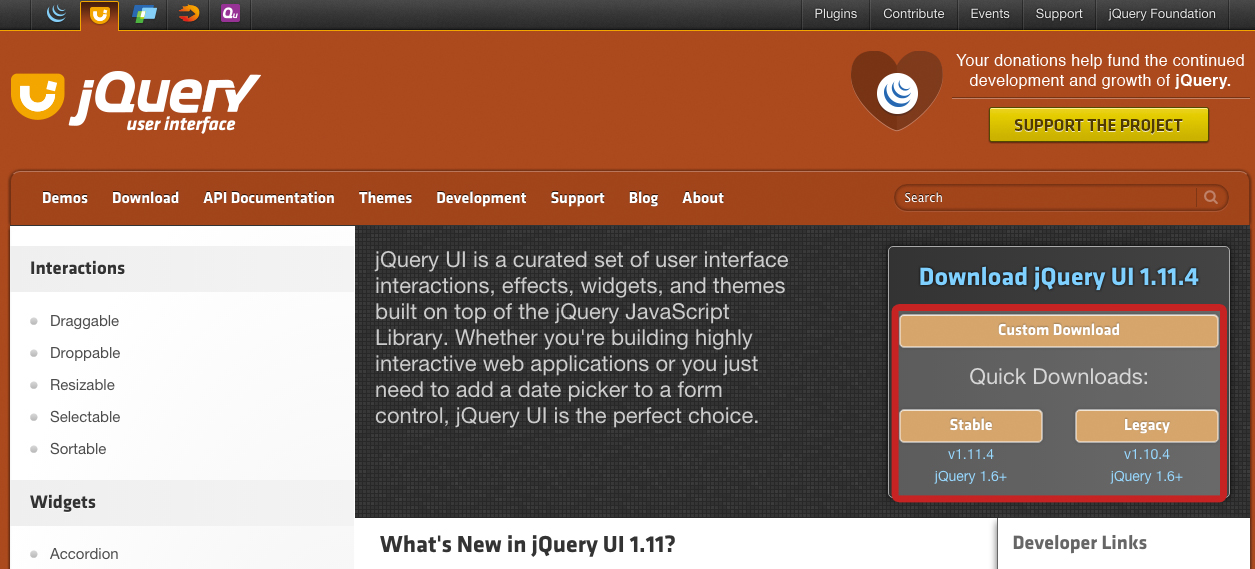Caption:

This detailed screenshot highlights the homepage of the jQuery User Interface web app. The top navigation bar features tabs labeled "Plugins," "Contribute," "Events," "Support," and "jQuery Foundation." A prominent message beneath encourages donations to help fund the ongoing development and growth of jQuery, accompanied by a yellow "Support the Project" button.

A secondary navigation menu includes "Demos," "Download," "API Documentation," "Themes," "Development," "Support," "Blog," and "About," alongside a search bar. The left sidebar lists interactive features such as "Draggable," "Droppable," "Resizable," "Selectable," and "Sortable," as well as widgets like "Accordion."

Central to the page is the jQuery UI logo and a comprehensive description: "jQuery UI is a curated set of user interface interactions, effects, widgets, and themes built on top of the jQuery JavaScript library. Whether you're building highly interactive web applications or you just need to add a date picker to a form control, jQuery UI is the perfect choice."

Highlighted in the middle of the page are download options for jQuery UI 1.11.4, including "Custom Download," "Quick Download," "Stable," and "Legacy," each enclosed in a red box, drawing the viewer's focus. The screenshot effectively captures the essential elements and usability features of the jQuery UI homepage.